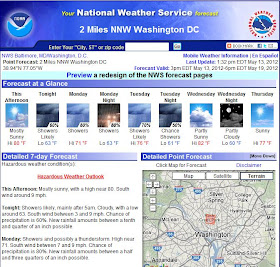This is a detailed screenshot of a redesigned National Weather Service (NWS) forecast webpage. The top section features a blue gradient background that transitions from dark blue on the left to almost white on the right. Prominently displayed at the top is the text "Your National Weather Service Forecasts" with the words "Your forecasts" highlighted in yellow, while the rest of the text is in white. Directly below this heading, there is a light blue bar spanning the width of the screenshot, containing the text "Two Miles NNW, Washington, D.C." 

Below the blue gradient section, the screenshot displays nine thumbnails in a grid pattern. The left side beneath these thumbnails contains a block of text, while the right side features a detailed map of Washington, D.C. The overall layout is a compact preview of the updated design for the NWS forecast pages, providing a clear and concise visual representation of local weather information.